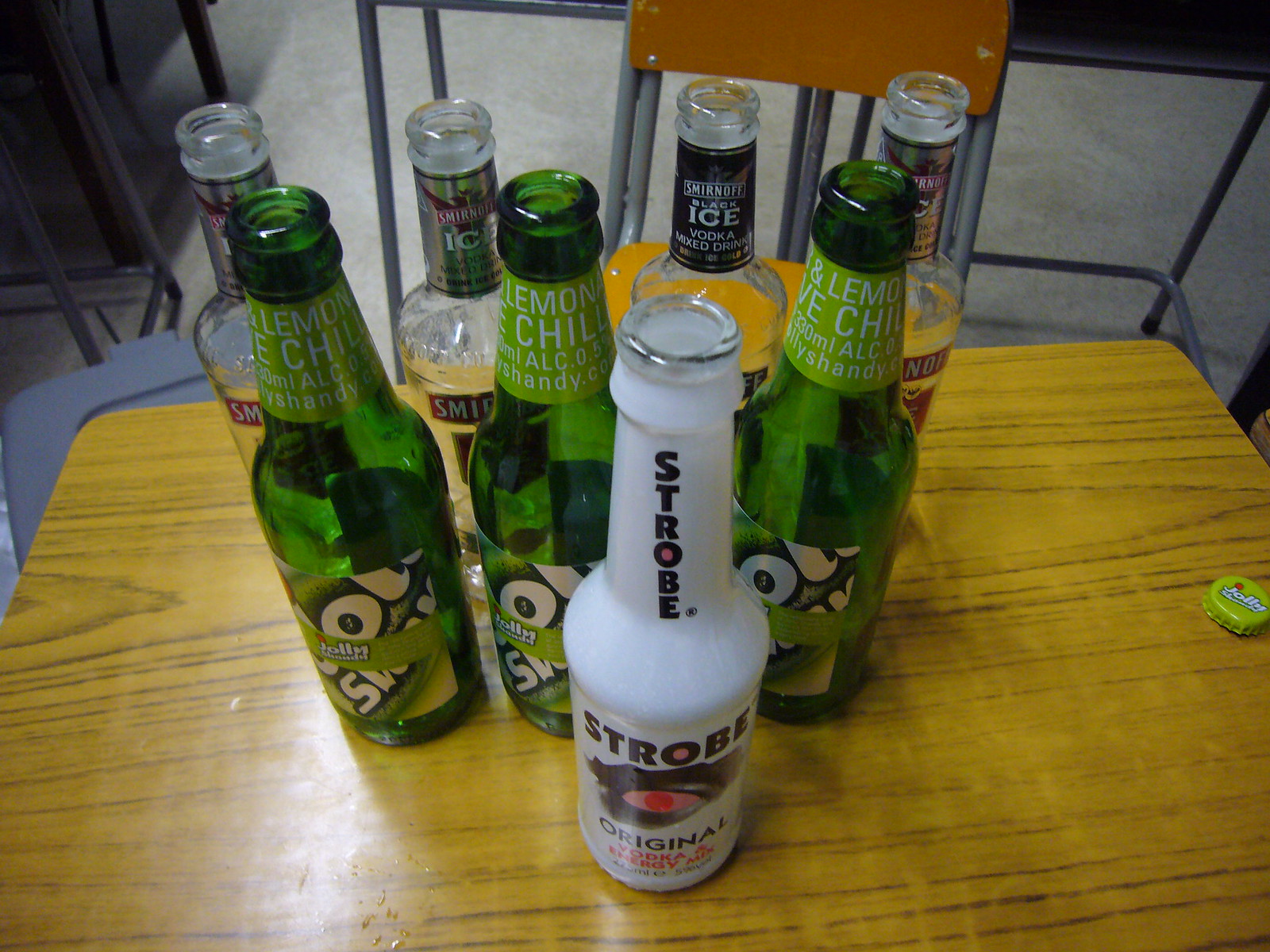The image features an array of eight empty alcoholic drink bottles arranged on a light brown, grainy wooden table, viewed slightly from above. In the immediate foreground stands a distinctive white bottle labeled "Strobe Original" in black letters, with a striking red-filled "O" and a red eye symbol on the label. Directly behind this are three green glass bottles, each marked "Lemon Chill" on a green and beige label. Further back are four clear bottles of Smirnoff Ice, recognizable by their black neck labels with white Smirnoff text and the iconic red Smirnoff rectangular label partially visible. The bottles are neatly aligned in a triangular formation. To the right on the table lies a lime green bottle cap inscribed with the word "JOLLY." In the background, a metal-framed chair with a brown high back and an orange seat is partially visible, complementing the orderly setup on the lightly colored wooden table.